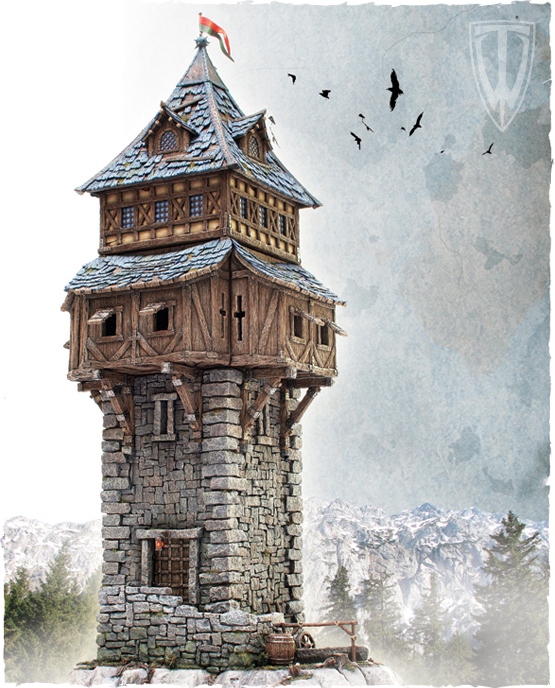The image is a detailed, old-style oil painting, evoking a European setting. Dominating the foreground is a tall, narrow tower with distinct architectural features. The base of the tower is constructed from gray stone, providing a solid foundation that supports the upper wooden section, which is designed in a Tudor style with light brown timber and shingled elements. The topmost section showcases dormer windows and is capped with a pyramid-type roof, sporting a red and white flag. The tower stretches upward with an elongated, rectangular form, featuring grates on the windows and possibly internal stairs ascending through its three levels. Behind the tower, the scenery transitions to a wintry background with snow-covered mountains and a stand of six or seven pine trees. The sky is overcast with gray clouds, adding to the somber mood of the scene. Black birds, possibly crows, fly ominously above the tower. A watermark, a stylized shield containing the initials "TW," is visible in the upper right corner, although the artist remains unidentified. Overall, the painting exudes a fantastical, almost folkloric quality reminiscent of European myths like the tale of Baba Yaga.